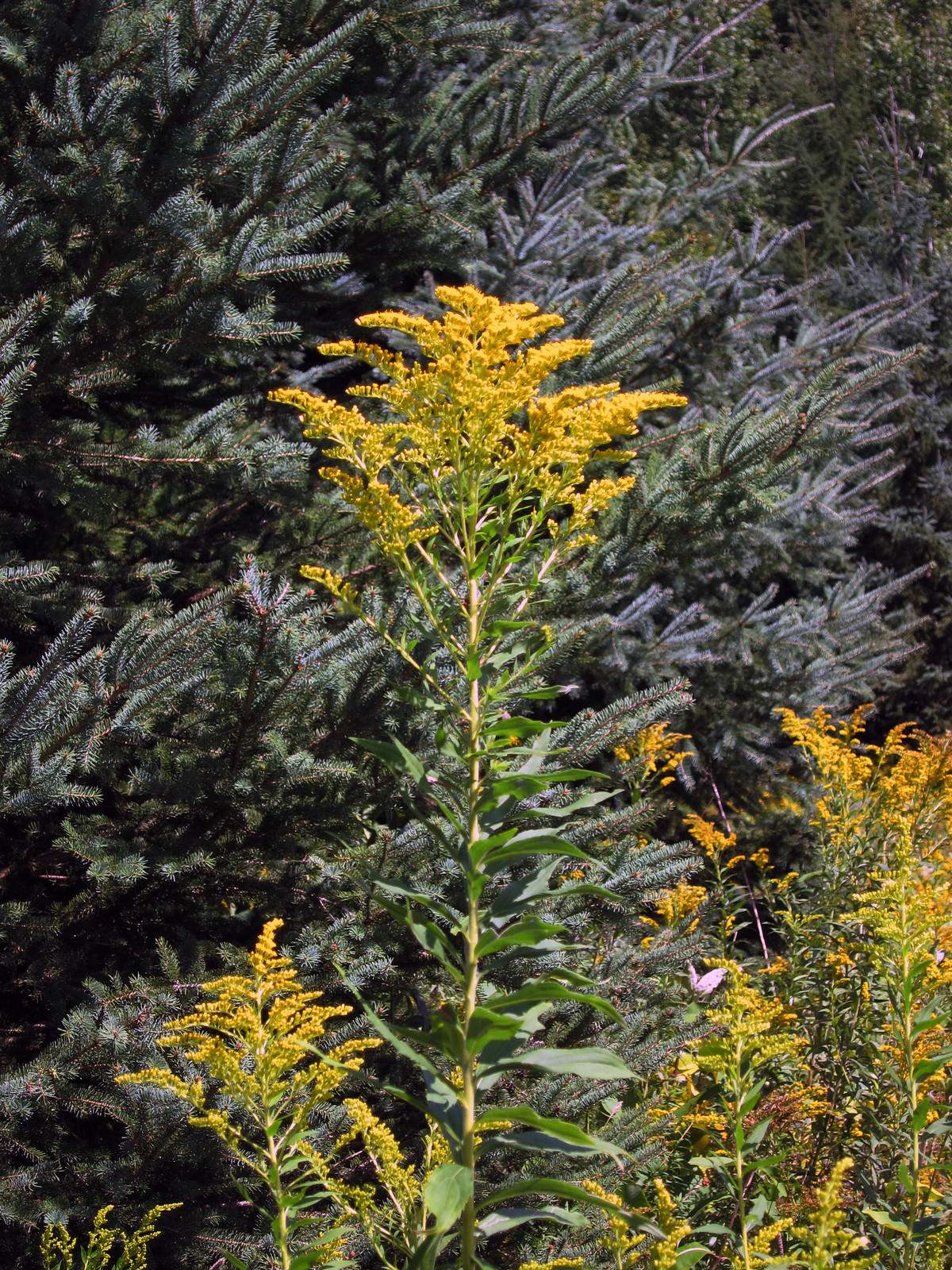This vibrant, high-resolution photograph captures a stunning display of nature's beauty. The foreground prominently features several tall, slender wildflowers with green stems and leaves, crowned with striking yellow blossoms. Among these plants, the one in the middle stands out noticeably, appearing significantly taller than the others, likely due to camera perspective. Surrounding this central wildflower, more green foliage and yellow accents can be seen, adding depth to the scene.

In the background, a lush tapestry of greenery is formed by numerous large pine trees or possibly ferns, each characterized by their spiky green needles. Their dense boughs provide a rich, textured backdrop that complements the focal wildflowers. 

Adding to the photo's dynamic nature, a delicate butterfly or moth, with hues of pink and purple, rests on one of the plants at the bottom right, lending an additional element of life and color to the image. This photograph is a detailed and colorful celebration of the intricate beauty found in a natural setting.